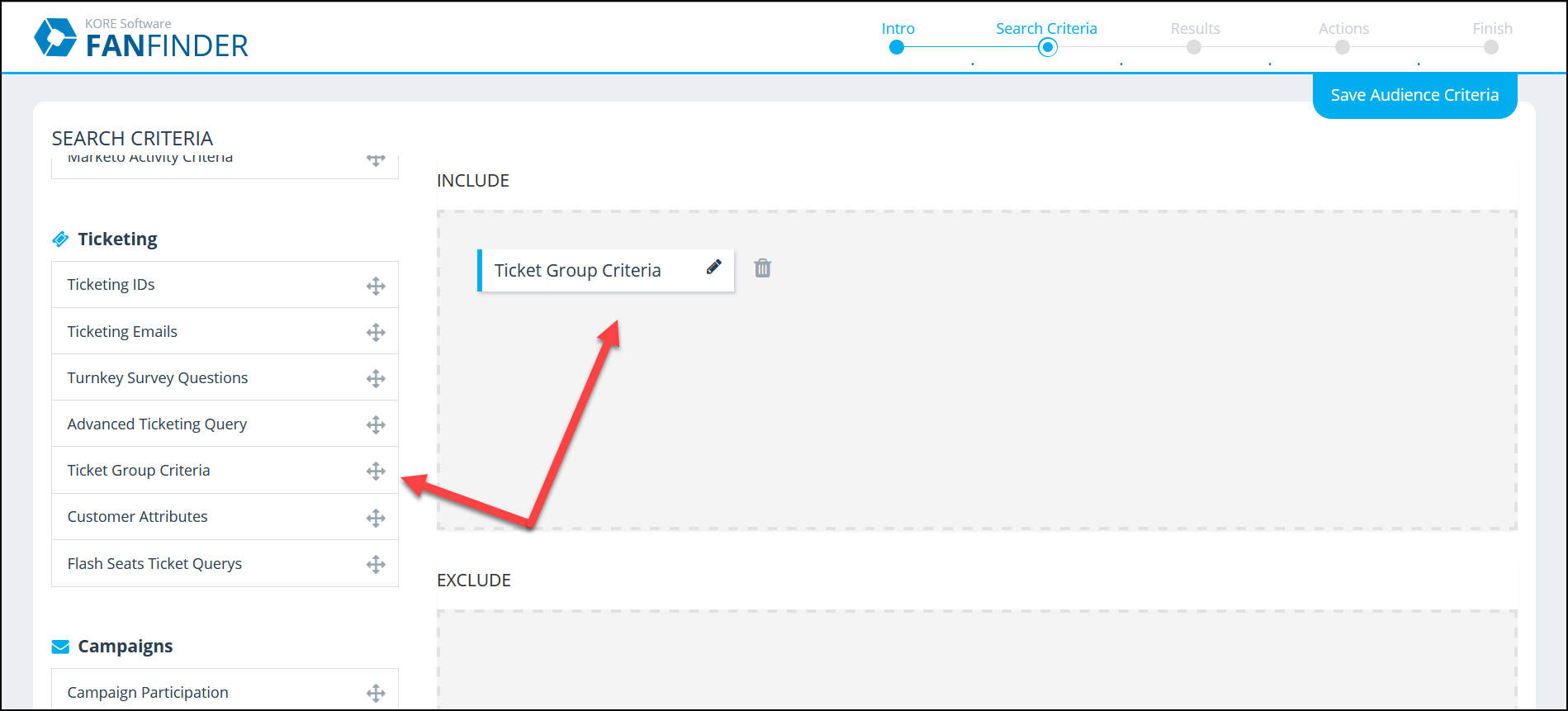A screenshot of a website with a thin black outline features a detailed header at the top of the page. The header begins on the left with a blue hexagon containing three white lines and an off-kilter, rounded white square in the center. To its right, two lines of text are displayed. The top line is small, light gray, and spells "KORE" in all caps. Beneath it, in blue text with the word "FAN" bolded and "FINDER" not, reads "FANFINDER" also in all caps. The right portion of the header is dominated by a segmented line: the initial segment is blue, followed by three light gray segments. Each intersection of these segments is marked by circles of varying designs. The first circle is entirely blue, the second is a smaller blue circle with a thick white outline and a thin blue border, while the remaining circles are light gray.

Above each circle, text is displayed, reading from left to right: "INTRO" and "SEARCH CRITERIA" in blue text, and "RESULTS," "ACTIONS," and "FINISH" in light gray text. Beneath each stretch of the segmented line lies a tiny blue dot.

Following the header, a bright blue line spans the width of the page. On its right side, a bright blue tab with rounded bottom corners hangs down. It contains white text reading "SAVE AUDIENCE CRITERIA." The body of the page, beneath the bright blue line, shows a light gray background with a white pane overlaying it.